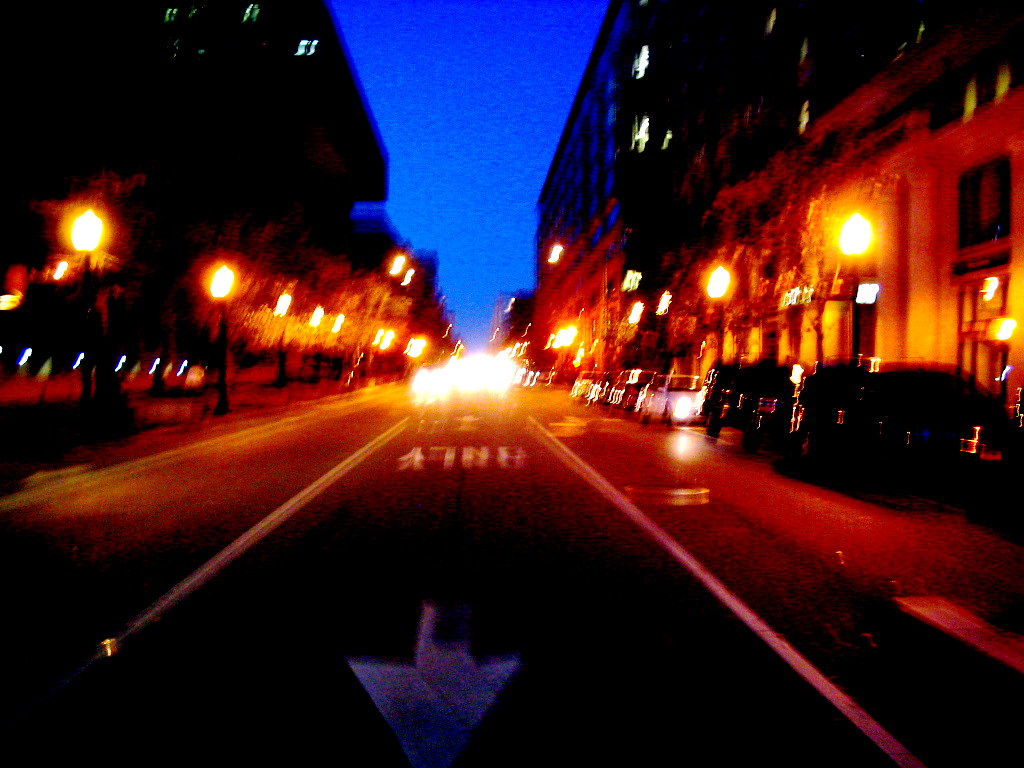This is a blurry nighttime photograph of a city street, possibly taken from a moving vehicle or a walking pedestrian. The perspective suggests the image was captured through the passenger side window. The street in the image is a one-way road, with visible markings including an arrow pointing towards the photographer and a sign saying "ONLY," indicating that traffic can only go straight. The street is flanked by buildings on both sides, some of which have lit windows. Streetlights and car headlights blend together, creating an overexposed effect, while a dark blue sky suggests either dusk or dawn. Cars are mostly parked on the right side of the street, with some cars’ headlights in the distance blending together. Additional elements such as light poles, possibly in a median, and trees are also visible, contributing to the urban ambiance of the scene. Overall, the photograph captures a lively but blurred snapshot of city life at a tranquil time of the day.